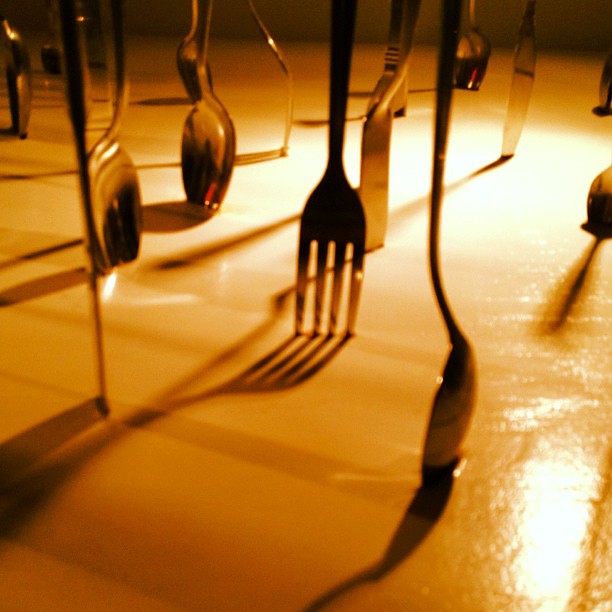In this image, we observe an array of cutlery, including spoons, forks, and butter knives, standing upright, inserted into the surface of what appears to be a wooden table with a glazed, light brown to mustard-colored finish. The arrangement features a prominent spoon in the forefront, standing on its bowl, while a fork stands balanced on its tines, and a knife rests upright on its blade. All the utensils exhibit a dark bronze-like shimmer. The scene is illuminated by sunlight streaming through a nearby window, creating reflections on the polished table surface and casting subtle glows on the cutlery. Additional bronze-colored spoons and knives are seen in the background, uniformly spaced out, with a gray wall visible in the distance behind the table, enhancing the overall composition.